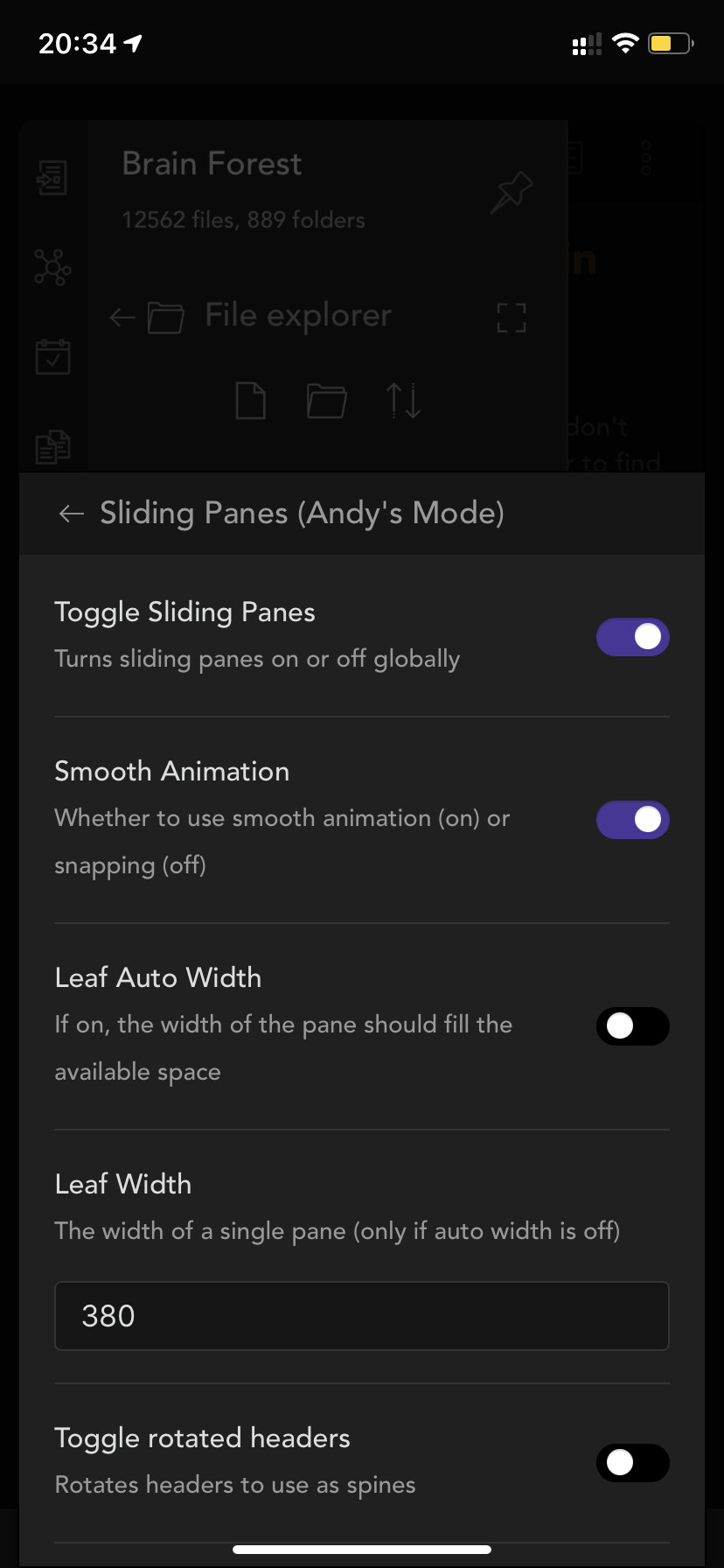A detailed screenshot from a phone set in dark mode. The device's display shows the time as 20:34, with full Wi-Fi strength and a half-charged battery indicated by a yellow icon. At the top, in faint letters, appears the name "Brian Forrest," with some barely readable text beneath it. The screenshot captures settings primarily focused on pane customization options. 

Here's a breakdown of these settings:
- **Toggle Sliding Panes:** This option, which is currently turned on, allows the user to enable or disable sliding panes globally.
- **Smooth Animation:** This setting, also activated, determines whether smooth animation should be used for swiping.
- **Leaf Auto Width:** This option, set to off, controls whether the pane's width should automatically fill the available space.
- **Leaf Width:** Here, the specific width of a single pane is adjusted to 380 since 'auto width' is disabled.
- **Toggle Rotated Headers:** This feature, which is switched off, controls whether headers should be rotated.

The entire display is set against a black background with white text, offering a stark contrast suitable for readability in low light conditions.